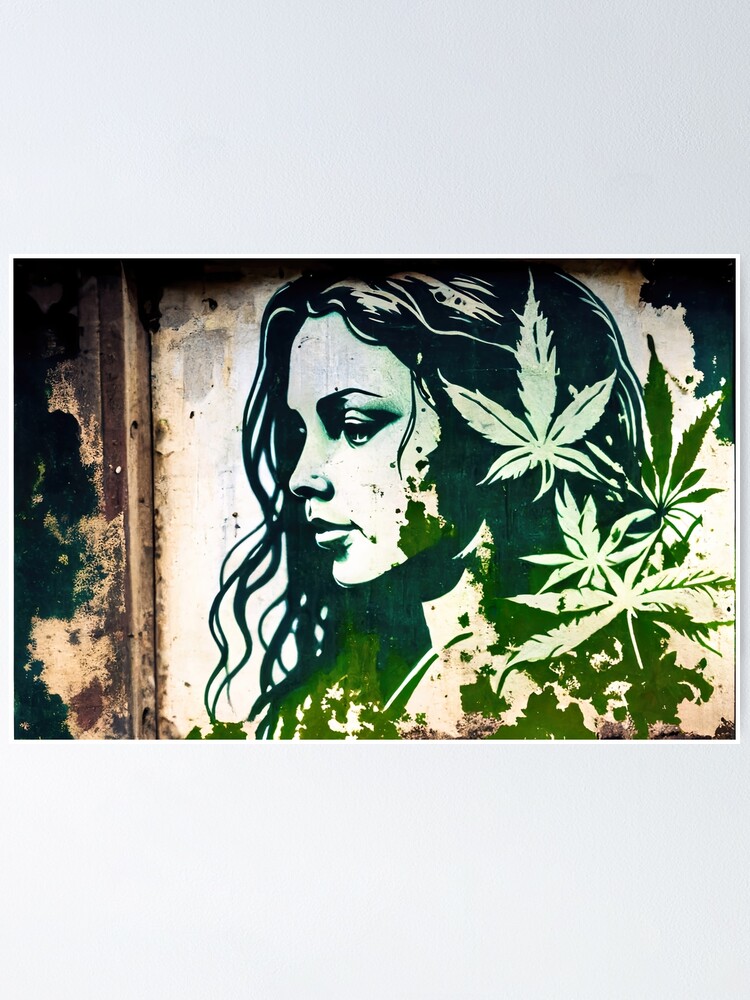This image is a detailed stylized painting, depicted in a photograph, showcasing a thoughtful side view of a woman's face and neck, as she looks to her right, our left. Her long, dark hair features several prominently placed marijuana leaves on the right side, contributing to the primary color palette of green, black, and creamy white. The woman's face is rendered in delicate shades with striking green tinges on her eyebrows and eyelashes, contrasting against the neutral white background. The background appears worn and textured, suggesting this could be a mural on an old, discolored wall, perhaps even a garage door with visible splotches and rust marks. This painting is a graceful blend of monochromatic elements with touches of green, capturing a serene and contemplative moment.